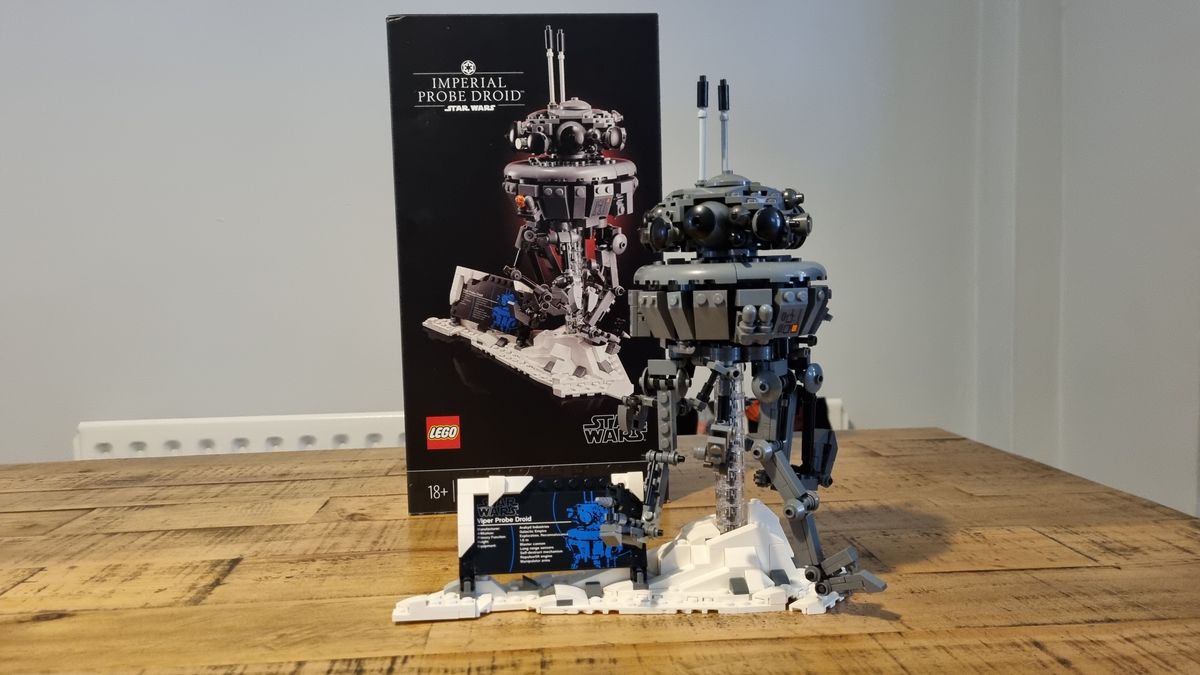The color landscape photograph showcases a meticulously constructed Lego Star Wars Imperial Probe Droid. The image highlights this impressive Lego creation, which stands right of center on a beige parquet wooden floor against a backdrop of white walls. The droid, notable for its elliptical head adorned with two silver antennas capped in black, features a segmented, cylindrical gray body with mechanical arms and legs. Positioned on a base designed to mimic Hoth's snowy landscape from "The Empire Strikes Back," the droid is accompanied by an informative placard to its left, though the details on it are not clearly legible.

Dominating the background is the droid's packaging, a large black box bearing a color photograph of the completed droid model, mirroring the assembled figure's sleek and accurate design. The box prominently displays "Imperial Probe Droid" in white text at the top left, with the Lego logo in red and white on the bottom left and the Star Wars logo on the bottom right. The photograph captures the striking realism and detailed craftsmanship of the Lego model, providing a side-by-side comparison with the box art, emphasizing the remarkable accuracy and scale of this cool collectible for Star Wars enthusiasts.